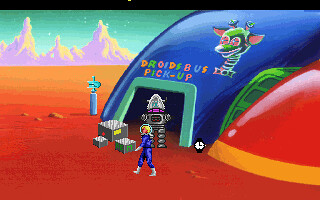This image is a screenshot from an old, vividly colored video game set on a desert-like, orange planet. In the foreground, a small figure, resembling a blonde female character, is dressed in a blue spacesuit with white gloves and boots, walking across the landscape. The background features a blue dome structure with an aquamarine rectangular entrance labeled "Droids Are Us Pick Up." Near this blue dome, there's a red dome and between them, a small wristwatch is visible on the ground. A quirky, green space giraffe is displayed above the "Droids Are Us" sign. Another character in a blue spacesuit with a clear helmet stands in front of the blue dome, suggesting a busy, adventurous atmosphere. The scene is animated by a backdrop of mountains and sky, with various red elements accentuating the ground, adding to the game’s vibrant and dynamic aesthetic.